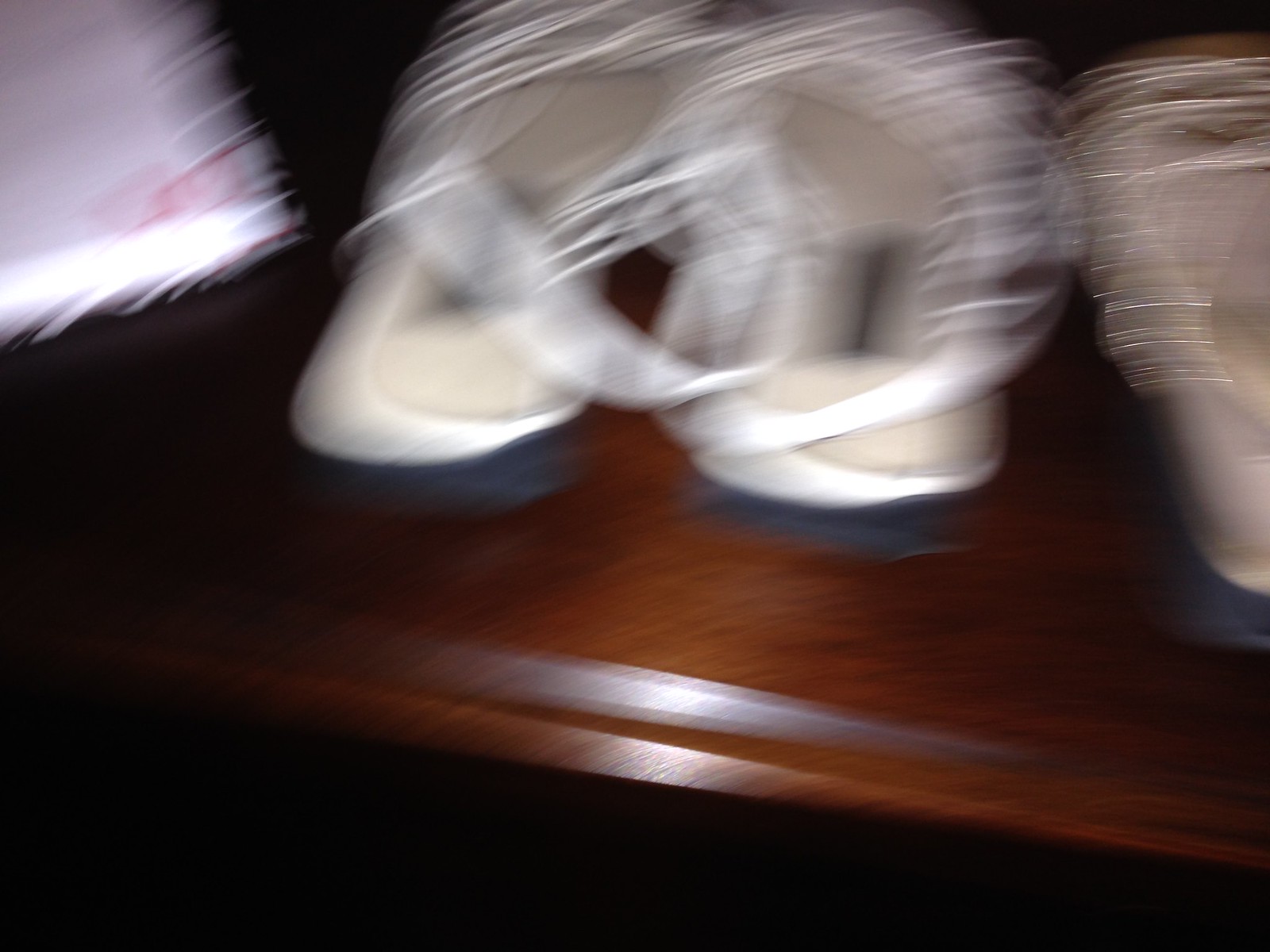In this rather blurry image, there's a wooden platform with shades of brown resembling walnut. At the center, a pair of high-end women's sandals with white straps, beige soles, and a black bottom is prominently displayed. To the right, there's a single gold sandal with similar high-end design. To the left of the white sandals, a pink object can be discerned, which might be a book or a purse with a white cover. The background beneath the wooden platform appears to be black.